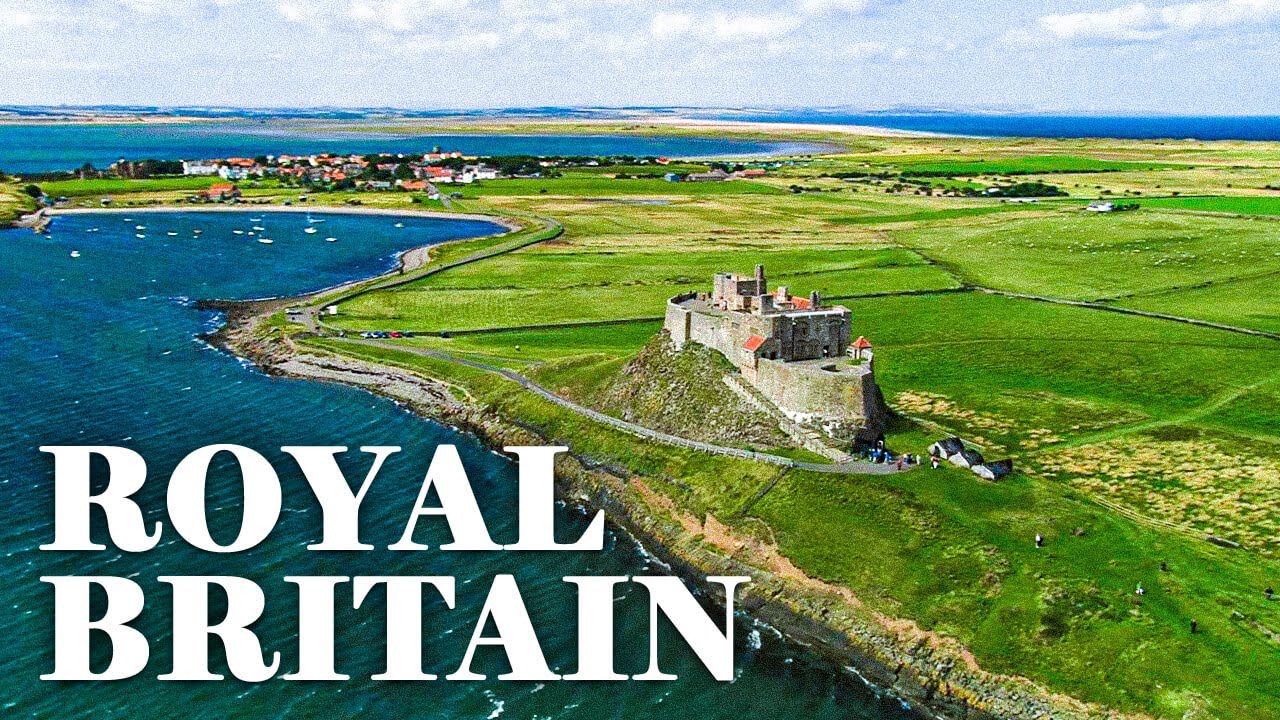The image displays an aerial view of a small, ancient fortified castle situated by a winding shoreline, surrounded by lush green fields and intersecting roads leading through the picturesque countryside. In the distance, a quaint village of creamish-gray houses with black rooftops is visible. The castle, which features distinctive orange, triangular shapes, is set against a backdrop of either a river or lake, with some orange-hued rocks lining the shore. A staircase and a road ascend from the parking lot toward the castle, indicating pathways for visitors. The daytime scene is illuminated by sunlight, casting visible shadows beneath a sky filled with clouds. In the bottom left corner, large yellow capitalized letters spell out "Royal Britain," suggesting this could be the cover of a book, a postcard, or the introduction to a television program, emphasizing the royal heritage associated with the castle and its scenic coastal surroundings.